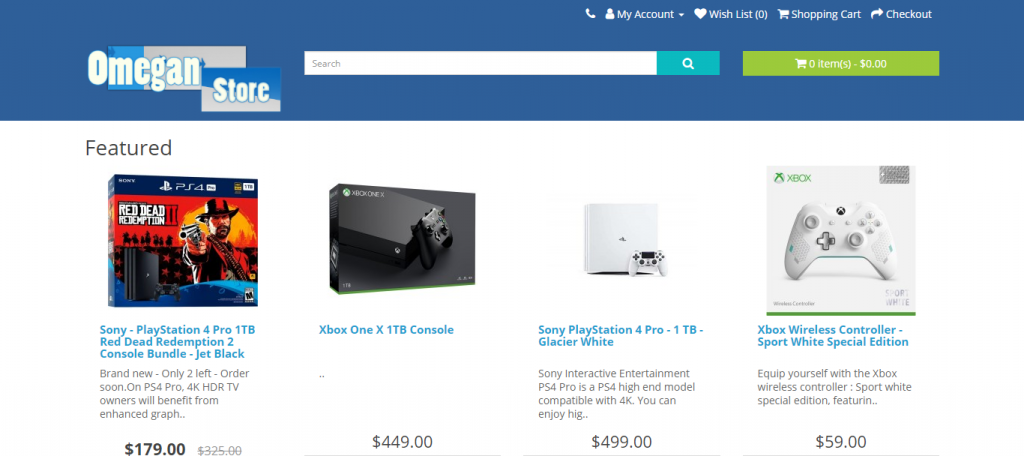The image depicts the homepage of the Omega Store, prominently featuring the store's name in the upper left corner within a thick blue strip that stretches horizontally across the top of the page. The 'Omega Store' logo is rendered in white with a blue outline, set against a background of blue and gray rectangular shapes.

In the center of this strip, there's a search field with the placeholder text "search" in gray and a teal button with a white search icon adjacent to it. To the right of the search bar, a bright chartreuse display indicates "0 items" with a cart icon, and "0.00" in white text.

The upper right corner, beginning from the middle, features several elements: a phone icon followed by the text "My Account" with a dropdown menu, a heart icon labeled "Wish List" with a "0" in parentheses next to it, and links to the shopping cart and checkout.

Below the navigation bar, the page showcases the "Featured" section, displaying four items in a row. The first item is the "Sony PlayStation 4 Pro 1TB Red Dead Redemption 2 Console Bundle - Jet Black," priced at $179, marked down from $325. The adjacent item is an "Xbox One X 1TB Console" listed at $449. The third item is a "Sony PlayStation 4 Pro 1TB - Glacier White," priced at $499.